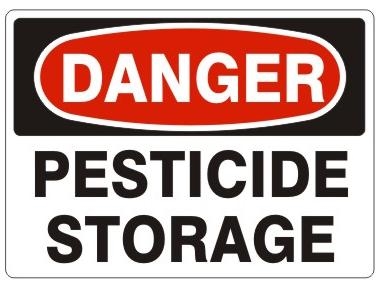The image depicts a rectangular warning sign, typically found in workplaces, made of metal or thick plastic. The sign features a clear, bold design intended for high visibility and comprehension. At the top of the sign, there is a large black rectangle with a prominent red oval inside it, containing the word "DANGER" in bold white letters. This section is set against a white backdrop with beveled edges, ensuring the sign has no sharp corners. Below this, the white background continues with the words "PESTICIDE STORAGE" prominently displayed in large, black, bold letters. The overall design of the sign, with its distinct red, black, and white color scheme, serves to effectively alert individuals to the presence of pesticide storage, emphasizing safety and awareness.